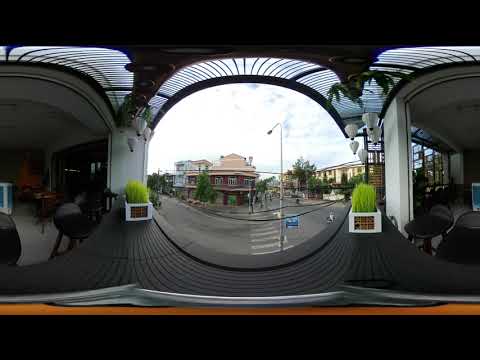This panoramic, 360-degree photograph captures a vibrant and eclectic urban scene from inside a quaint little café. The café features some black chairs and tables, with a mix of red wood-colored furniture scattered throughout. Lights and various decorations hang from above, adding to the cozy and inviting atmosphere. 

As the image pans outward from the café, you can see a bustling city intersection framed by black pavers and a metal awning. The intersection features a well-marked crosswalk and a light pole emerging from the pavers. To the left and right of this central view are planters filled with green shrubbery.

To the left side of the image, a red building with a light sand-colored roof is prominently featured, alongside a white building and a darker one in the background. On the right side, there is a cream-colored building partially obscured by a green tree.

The front of the café is adorned with a charming planter box filled with vibrant plants, adding a touch of greenery to the scene. Ornate and pretty lights enhance the storefront's welcoming appearance. Beyond the immediate foreground, the vibrant city blocks and meticulously planned neighborhood suggest a tourist-friendly area with shops lining the streets. The sky above is bright and filled with clouds, casting a soft light over the entire setting, contributing to the overall picturesque and lively ambiance.